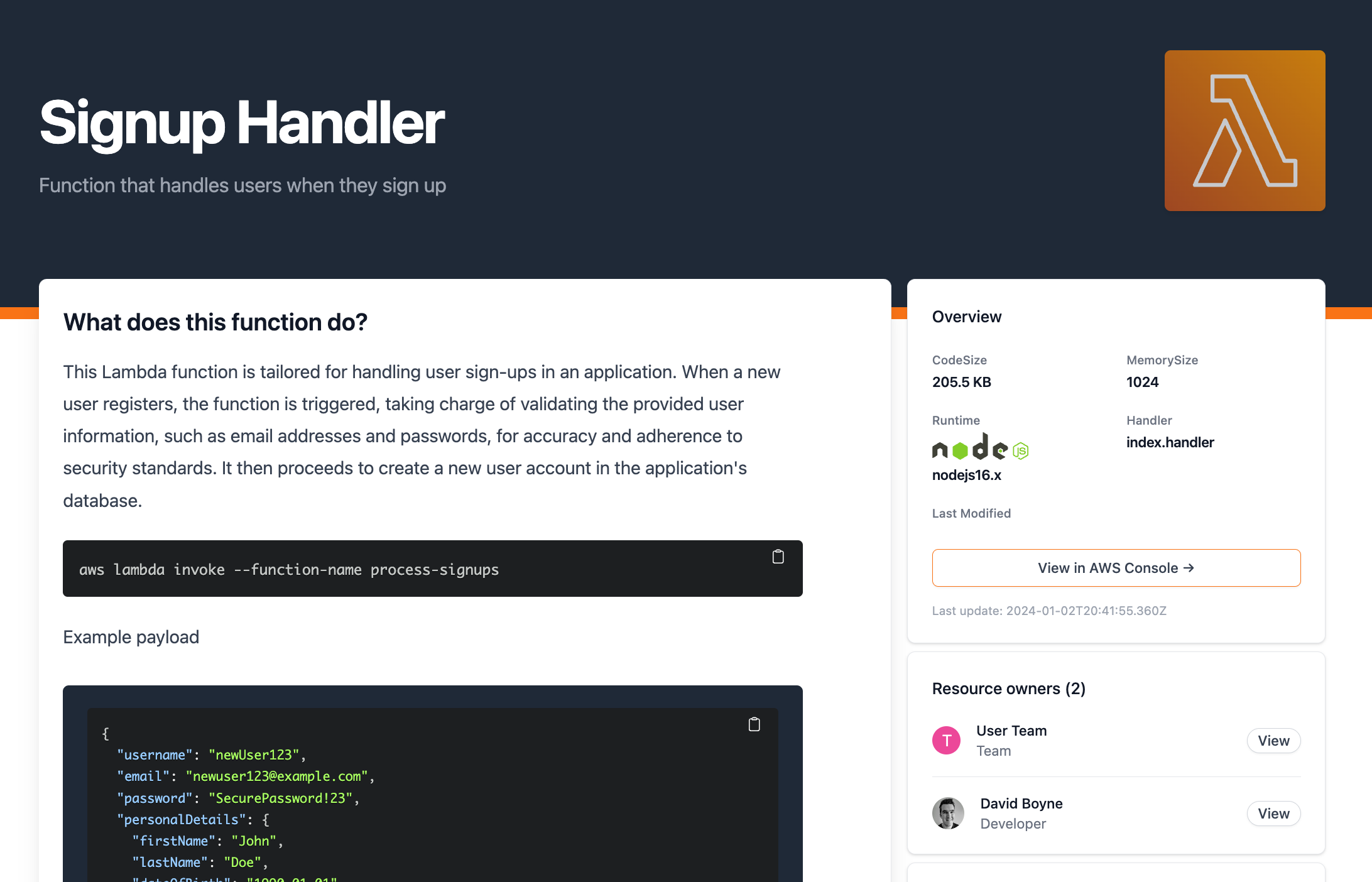The image displays a web page showcasing a "signup handler function" designed for managing user registrations in an application. This Lambda function is meticulously crafted to activate whenever a user signs up, performing crucial tasks such as validating user information including email addresses and passwords. Programmers frequently utilize this type of coding function, which leverages pre-written code libraries and packages. The specific function shown is accompanied by a snippet of its code detailing variables for username and password, among other elements. On the right side of the page, additional information is provided, including the file size, the function's name (referred to as "handler"), runtime environment indicated as "Node.js," and resource owners, which lists two individuals.